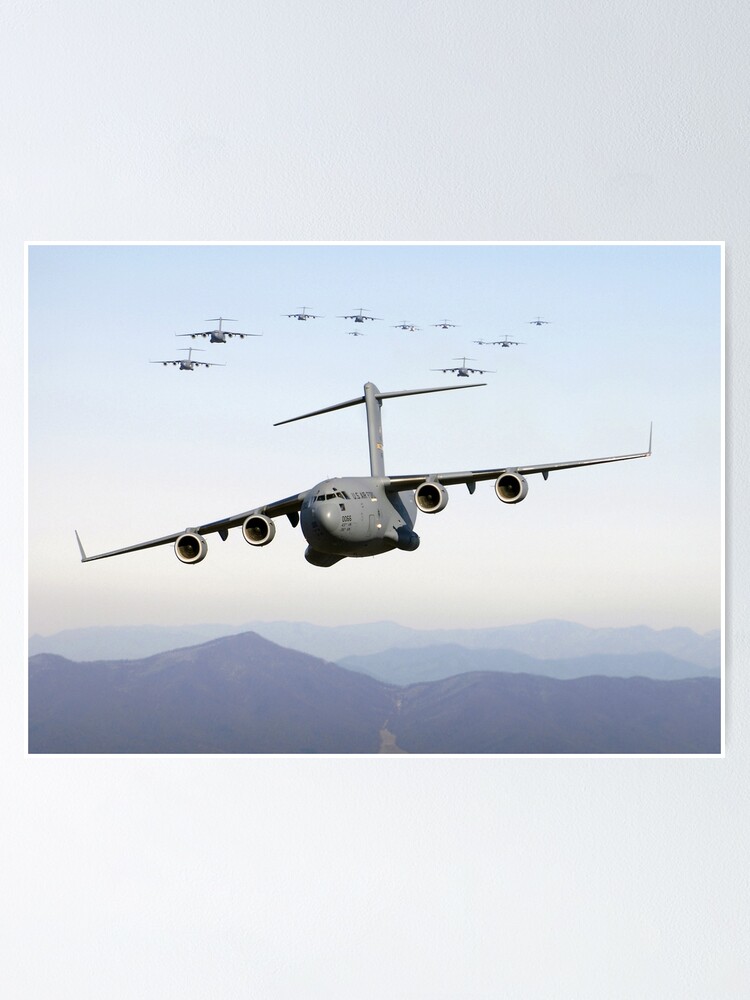In the center of the image is a photograph of several military airplanes, prominently featuring a large grey bomber in the foreground with four engines—two on each wing. The scene is set against a background of a light blue sky that fades to white and grey, with dark, fuzzy mountains beneath, suggesting high elevation and distant fog. The primary aircraft, highlighted and slightly tilted to the left, is flanked by a considerable number of identical bombers, 12 in total, all flying in the same direction and perspective, creating the illusion of a vast formation. The meticulous details include additional smaller airplanes trailing in the distance, and the stark, vertical tail spars of the bombers add to their imposing presence. The entire image, evocative of a mid-air military exercise, is placed against a plain white or greyish painted wall, reminiscent of a poster or print mock-up.